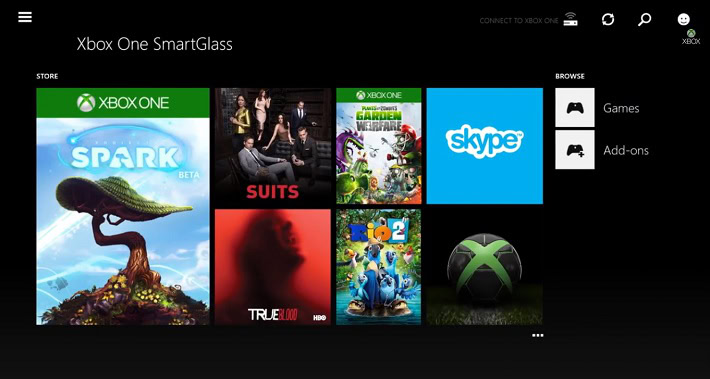Screenshot from a website featuring a sleek black background layout. In the top left corner, there is a square icon composed of three white horizontal lines, often referred to as a "hamburger menu." On the top right, there's a text label that reads "Connect to Xbox One." Accompanying this label are four icons: an Xbox One console icon, a circular icon, a magnifying glass icon, and a smiley face icon. 

Beneath the smiley face icon, a cluster of icons and text is displayed. The first icon in this cluster is the Xbox logo, depicted as a white circle with a green "X" inside. Directly below this icon, the word "Xbox" appears in white letters. Following this, a list of items is presented: "Xbox One SmartGlass," "Store," "Xbox One Spark Beta," "Suits," "True Blood," "Plants vs. Zombies Garden Warfare," "Rio 2," "Skype," and another Xbox logo, this time decorated on a soccer ball. On the right side, the options "Browse Games" and "Add-ons" are available.

The image has a landscape orientation, being wider than it is tall, and contains no people, animals, birds, automobiles, buildings, motorcycles, helicopters, airplanes, or food.